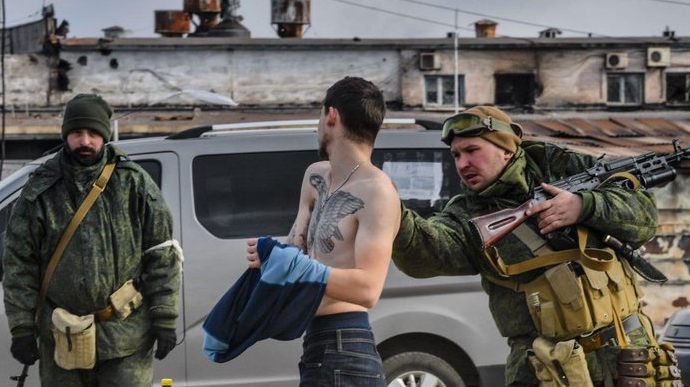The image depicts a tense scene at a war zone checkpoint. At the center, a shirtless, light-skinned man with a tanned complexion stands, displaying a large tattoo of a bird across his chest. Surrounding him are two heavily armed soldiers clad in green military jackets and extensive gear. The soldier on the right, who has goggles perched on his forehead, clutches a massive weapon and examines the man's back intently. Behind the group is a stationary gray van, set against a backdrop of small, industrial-looking buildings with air conditioning units and windows, suggesting a gritty, utilitarian environment. The soldiers' vigilant stance and the man's stripped state suggest a scenario where he is being scrutinized as a suspicious person or possibly a prisoner of war.